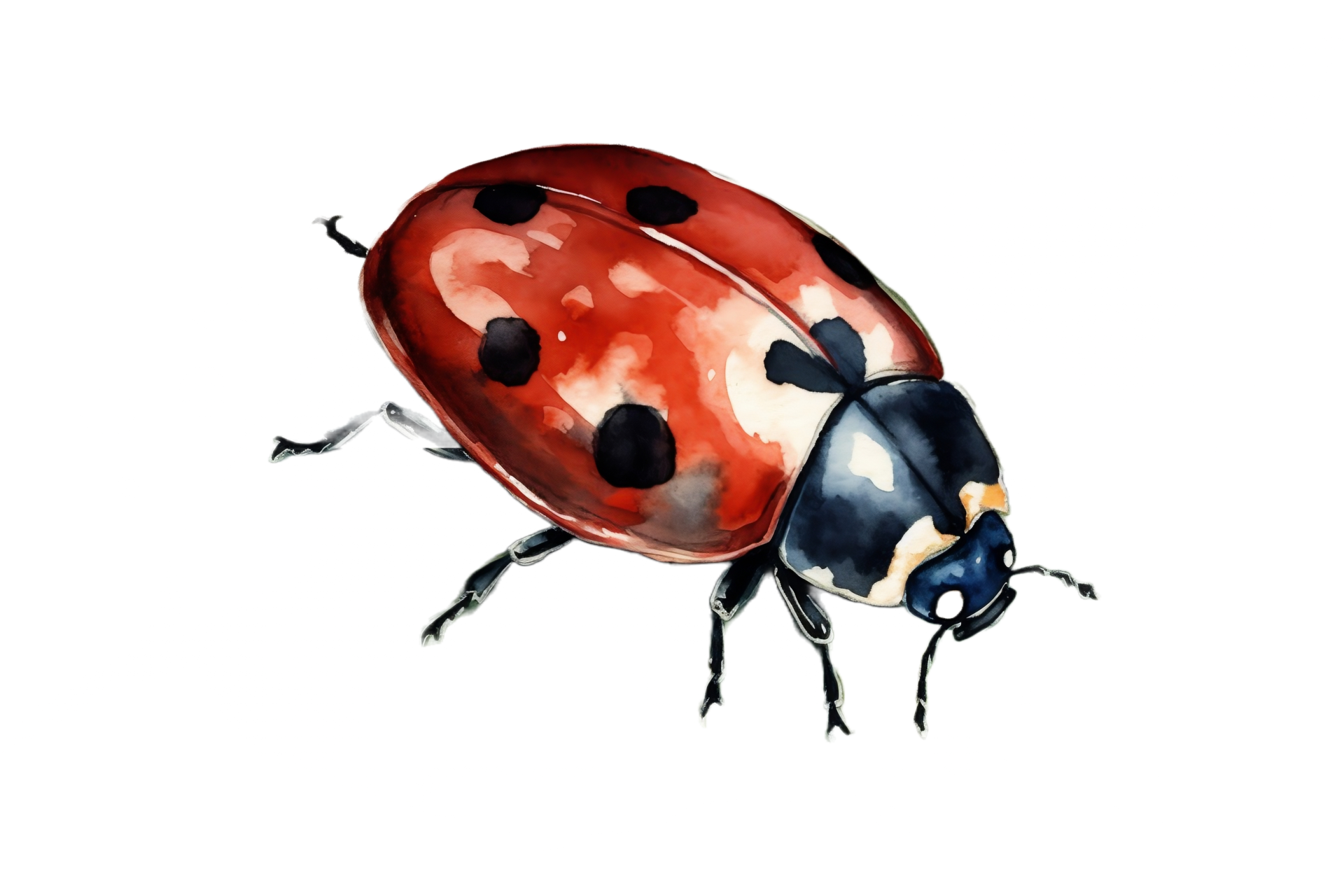This detailed illustration of a ladybug presents the insect against a stark white background, emphasizing the vibrant colors and intricate details of its anatomy. The ladybug's elliptical shell is a striking red, adorned with round black spots, and the depiction suggests highlights that create the illusion of light reflecting off its surface. The head is predominantly black, featuring white eyes and two prominent antennae extending out from beneath the eyes. A distinctive cream to yellowish neck strip separates the red shell from the black head. The insect is front-facing, showing its six legs, which are primarily black with hints of gray. The drawing captures the ladybug’s realistic anatomy and coloration, giving it a lifelike presence while maintaining an illustrative style.